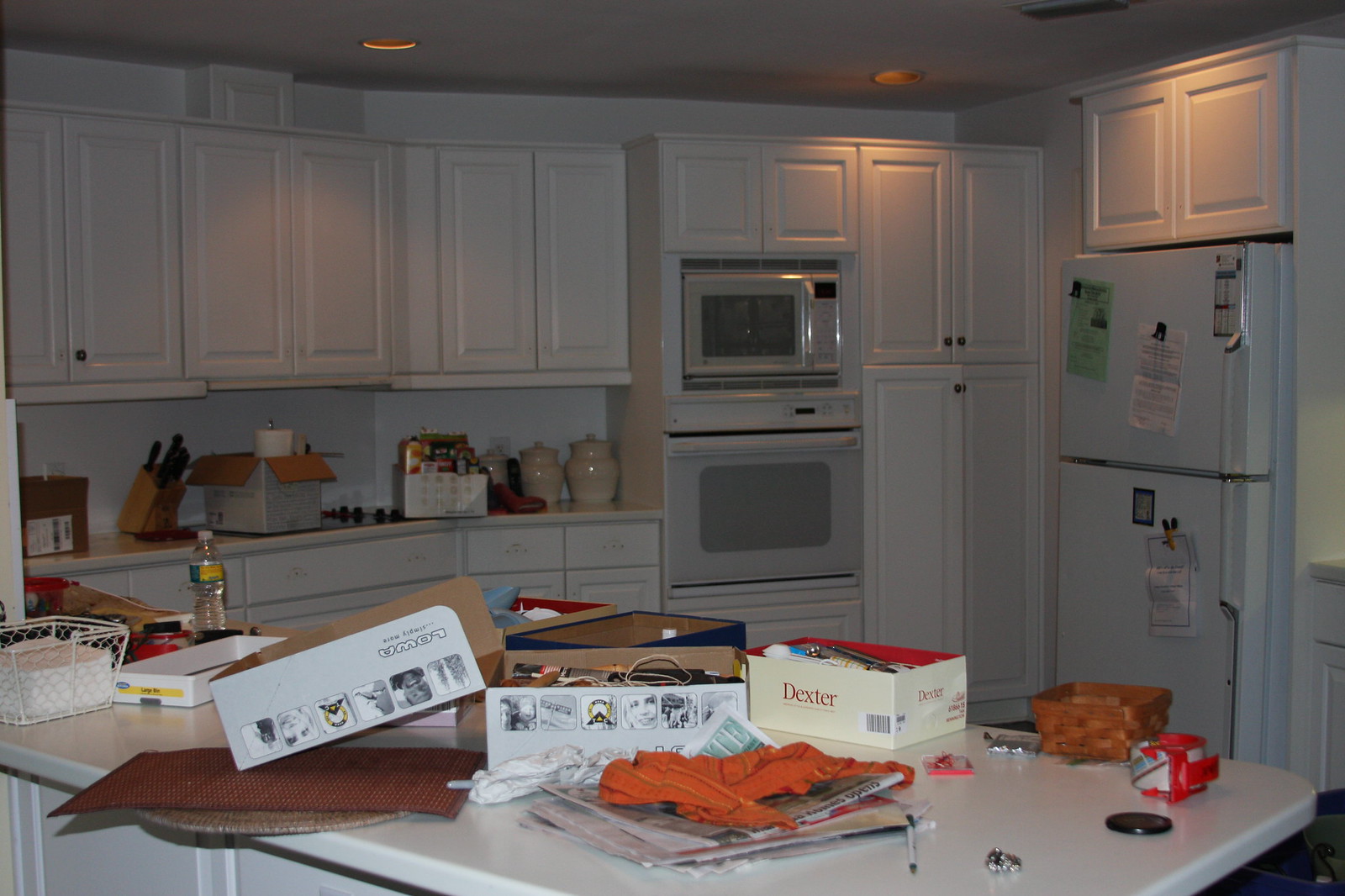The image depicts a contemporary kitchen characterized by its pristine white walls and matching white cabinets. A white refrigerator seamlessly blends into the background, enhancing the kitchen's clean and minimalist aesthetic. Contrasting the white elements, a rich brown countertop runs along the wall, providing a warm visual balance.

The kitchen features an island-style layout, central to which is a rectangular island table with elegantly curved edges, also in white. This island serves as a focal point and workspace and is adorned with various items. To the right side of the table, a roll of cellophane tape is visible. Adjacent to this, there's a small wooden basket, displaying a natural texture.

A white box labeled "Dexter" in bold red text stands out among the assortment of items. There are also several other boxes of differing colors, adding a splash of visual interest, as well as a piece of newspaper partially covered by an orange napkin. Two place mats are arranged on the island, suggesting spots for dining or working, and a sleek metal wire basket adds a touch of modern utility to the space. The overall composition of the kitchen is both functional and visually cohesive, reflecting a blend of simplicity and style.